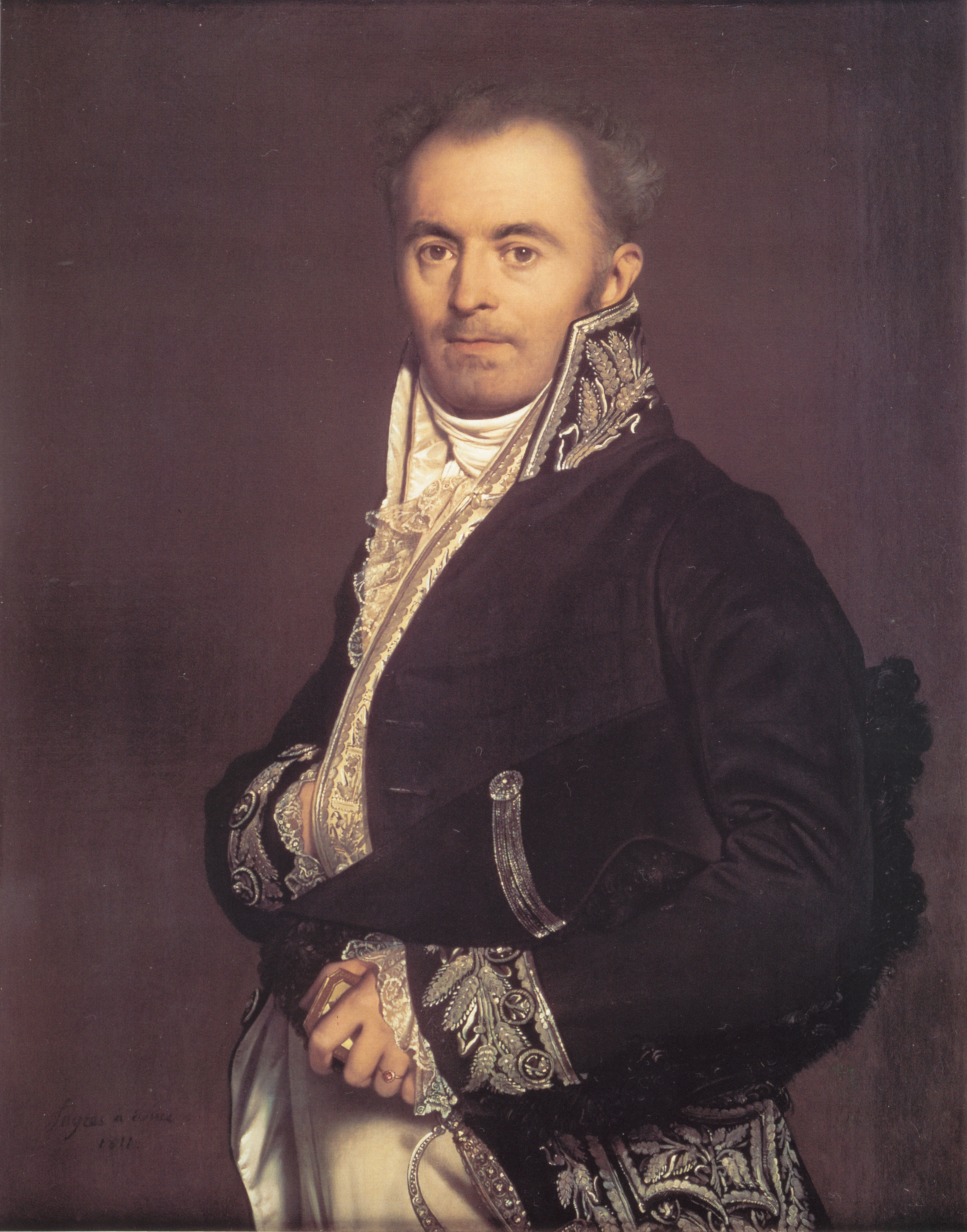This detailed painting, dated 1812, captures a regal and serious-looking gentleman, possibly a royal or military figure. He appears middle-aged, with fair skin, dark grayish hair with a high forehead, and a bit of scraggly stubble on his mostly clean-shaven face. His hairline is notably receded, featuring a slight widow's peak. The background is a dark purple wall, enhancing the viewer's focus on the subject.

He is posed with his body pointing towards the left but looking straight ahead, almost over the viewer's shoulder. Clad in an elegant, navy-blue long coat adorned with gilded designs, silver, and golden patterns, he evokes a sense of nobility. Underneath, he wears a high-neck, white brocade shirt that adds to his distinguished appearance. The sleeves and side pockets of his coat also feature white brocade details. 

In terms of accessories, his left hand carries a sword's handle, while the lower end of the saber rests by his leg, indicating his militaristic background. There is some ambiguity about him clutching a box or hat with a silver band under his arm. A signet ring gleams on the fourth finger of his left hand, while his right hand is tucked inside the lapel of his jacket, adding to his imposing stance. Completing his attire, he is seen in off-white trousers, contributing to a coherent and regal appearance.